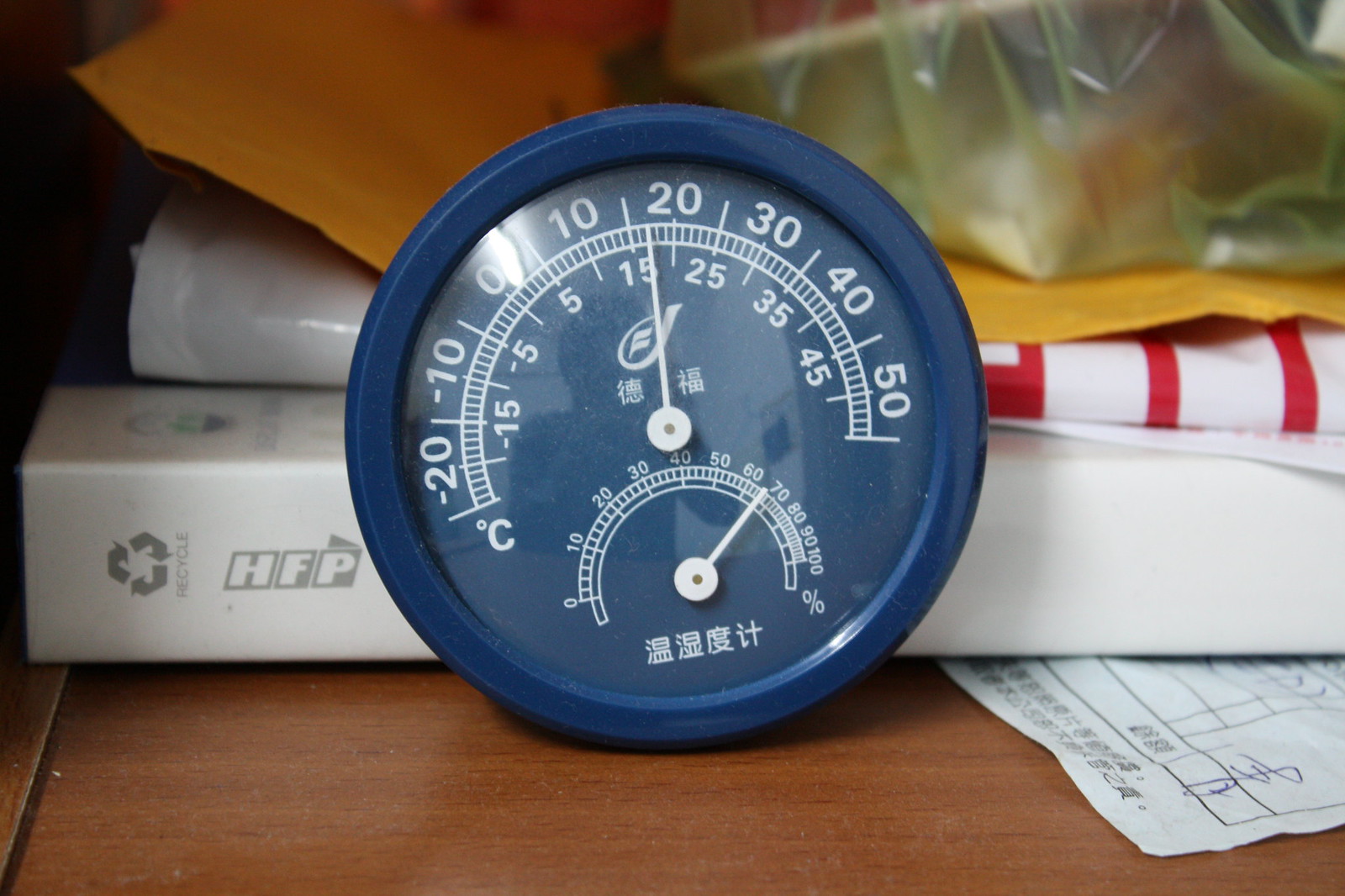The image features a round, blue thermometer with a built-in moisture gauge at the bottom. The thermometer resembles a small clock, encased in a translucent plastic cover. The blue face of the device displays white lines and numbers, ranging from -20 to 50 degrees. A thin white hand points to the temperature on the scale. In the center, there is an "F" and a sideways raindrop icon, accompanied by characters from an unrecognized language.

Below the main temperature scale, there is a smaller numerical line, bordered by additional characters that are equally unfamiliar. In total, there are six indistinguishable characters on the face of the thermometer. 

The device is positioned on a brown wooden surface, presumably a table or desk. In the background, there is a book and a chaotic pile of objects, including red, white, yellow, and translucent green plastic debris, along with a piece of paper that appears to be a receipt. The receipt features black print, boxes, lines, and what seems to be a signature with initials.